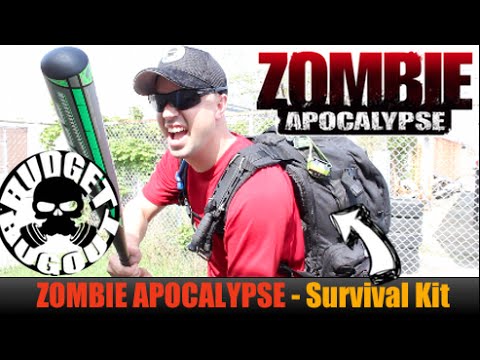The image is a YouTube thumbnail designed as an advertisement for a zombie apocalypse survival kit. It features a young white man with a bald head, wearing dark sunglasses and a gray hat, with a black tactical backpack. The man, dressed in a red t-shirt, holds a black and neon green baseball bat in an intimidating manner and gazes at the camera with a grimace-like expression. The scene is set against a blurred urban backdrop featuring a white fence and some greenery. 

Overlayed on the image, several vivid elements draw the viewer's attention: at the top right corner, bold red text reads "Zombie Apocalypse," and at the bottom of the image, in red and orange letters, it says "Zombie Apocalypse Survival Kit." Additionally, there is an icon in the lower left corner featuring a skull with a gas mask and the label "Budget Bug Out." An arrow points to the backpack, emphasizing the survival kit's contents. Black bands frame the top and bottom of the image, delineating its boundaries.